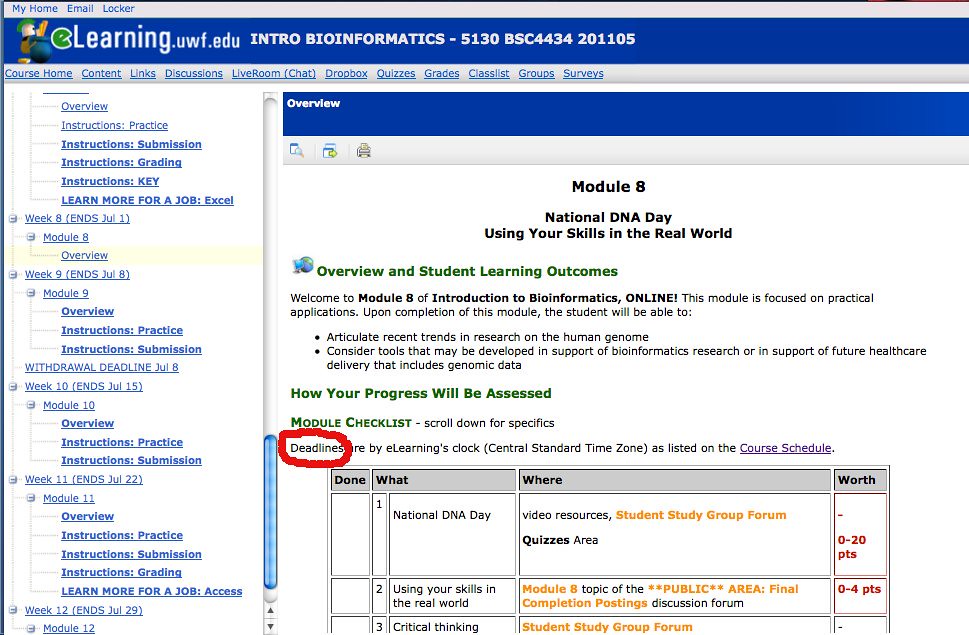This is a screenshot of a webpage from a bioinformatics course hosted on the University of West Florida's e-learning platform. At the very top of the page, in a section with a white background and blue font, the header displays "my home email and locker." Below this, there is a bright blue horizontal bar with the university's logo on the left side. Adjacent to the logo, which features a lowercase 'e' in green with a white border, the text "Learning.UWF.edu" is prominently displayed in white font.

Directly next to this, in bold white capital letters, it reads "INTRO BIOINFORMATICS - 5130 BSC4434 201105." Beneath this header bar are menu items listed horizontally, specifically: Home, Content, Links, Discussions, Live Room (with chat in parentheses), Dropbox, Quizzes, Grades, Class List, Groups, and Surveys.

Further down, spanning approximately two-thirds of the image and starting from a third of the way from the left edge, there is another horizontal bar labeled "Overview" in white font. 

In the main section of the image, which occupies the two-thirds space starting from a third to the right from the left edge, the title "MODULE 8" is centered at the top in bold black font. Below the title, the text "National DNA Day: Using Your Skills in the Real World" is also in bold black font. The subtitle "Overview and Student Learning Outcomes" is printed in green font.

The introductory content welcomes students to Module 8 of the Introduction to Bioinformatics online course, stating that the module focuses on practical applications. The intended student learning outcomes are listed in bullet points, which include:

- Articulate recent trends in research on the human genome.
- Consider tools that may be developed in support of bioinformatics research or future healthcare delivery that includes genomic data.

The section "How Your Progress Will Be Assessed" is in green font, followed by "Module Checklist" in black font, instructing students to scroll down for specifics. A red circle highlights the "Deadlines" section, which states, "Deadlines are eLearning's clock (Central Standard Time Zone) as listed on the course schedule," with "course schedule" in purple and underlined.

A schedule is provided below, organized in gray columns titled "Done," "What," "Where," and "Worth," with specific tasks listed underneath each column. On the left third of the image, a menu of instructional items appears vertically in blue font, listing options such as "Overview," "Instructions: Practice," "Instructions: Submission," "Instructions: Grading," "Instructions: Key," and "Learn More for a Job: Excel," among others.